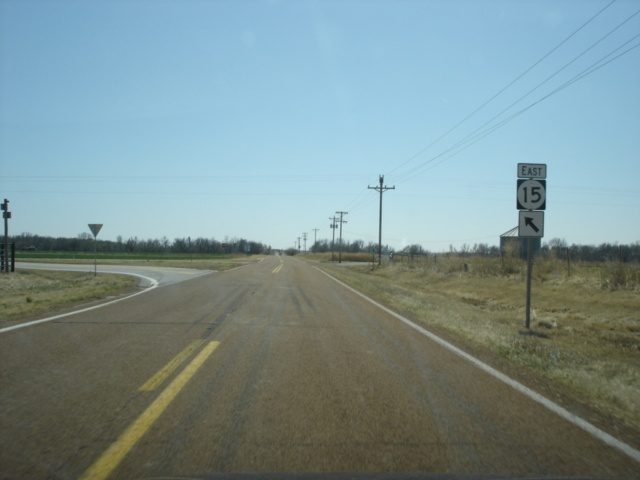This photograph captures a detailed view of a road stretching into the distance. The road itself is constructed of black asphalt with a slight brownish tint on the surface. It is bordered by solid white lines on both the right and left edges. Down the center of the road runs a combination of solid and dashed yellow lines, delineating traffic directions. Flanking the road are patches of low grass interspersed with areas of bare dirt; the grass shows a mix of green and white hues, suggesting varying stages of growth or seasonal change.

On the right side of the road, a sign mounted on a silver metal pole stands out. The sign features a two-part display: the top section is a black square with a white circle in the center, containing the number "15" in bold black digits, indicating a speed limit. Below this, a white rectangular sign has a black arrow pointing diagonally up to the left, likely indicating a turn or direction.

Additionally, lined along the road are telephone poles with wires strung between them, contributing to the rural atmosphere of the scene. On the left side of the image, another road branches off to the left. In the background to the left, rows of trees are visible, providing a leafy backdrop to the otherwise open setting.